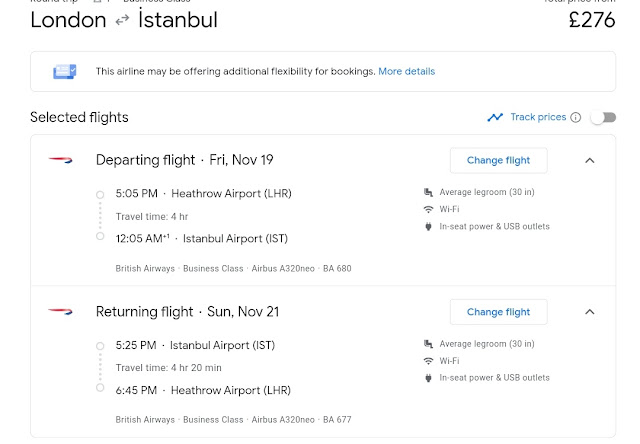**Screenshot of Airline Booking Details**

The image is a screenshot displaying flight booking details for an airline, set against a white background. At the top left, in large black letters, the route "London to Istanbul" is prominently featured, with arrows pointing left and right between the cities' names. 

To the right, the total price for the booking is displayed in bold, amounting to £276. Immediately below, there is a large box stating that "this airline may be offering additional flexibility for bookings." The words "more details" are hyperlinked in blue.

Beneath this box, on the left in bold gray font, is the label "Selected flights." On the far right, a toggle switch for "Track prices" is shown in the off position.

The subsequent section provides detailed flight information. The first segment outlines the departing flight, starting with the airline's logo on the left. Next to the logo is the text "Departing flight," followed by the date "Friday, November 19th." To the right of this is a clickable white box labeled "Change flight."

Below the departing flight details, it specifies the departure time as 5:05 PM from Heathrow Airport (LRH), with a white circle and dashed lines leading down to the arrival time at Istanbul Airport. 

The bottom section of the screenshot follows a similar format for the returning flight, featuring the airline logo on the left and "Returning flight" in large black letters, with the corresponding date to the right.